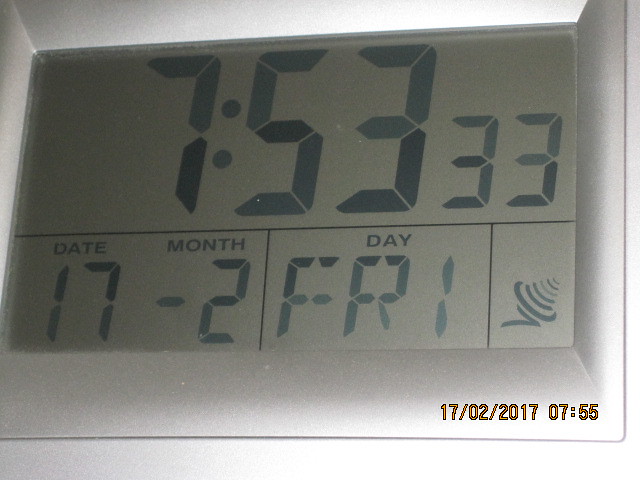An up-close image of an intricately designed alarm clock is centered in the frame. The inner components of the clock are a luxurious goldish pewter hue, set against a light gray background. Bold black numerals at the top of the clock display "7:53," accompanied by a smaller "33" underneath. Below this, a precise black line delineates the date section, which features the number "17" prominently. Adjacent to this, the word "month" is written in black, followed by a dash and the number "2." To the right, the word "day" is displayed, with "FRI" indicating that it is Friday. A small emblem nearby suggests the status of the alarm—whether it is on or off. At the bottom of the clock, the timestamp "17-02-2017-07:55" is displayed in vivid orange letters, adding a striking contrast to the overall design.